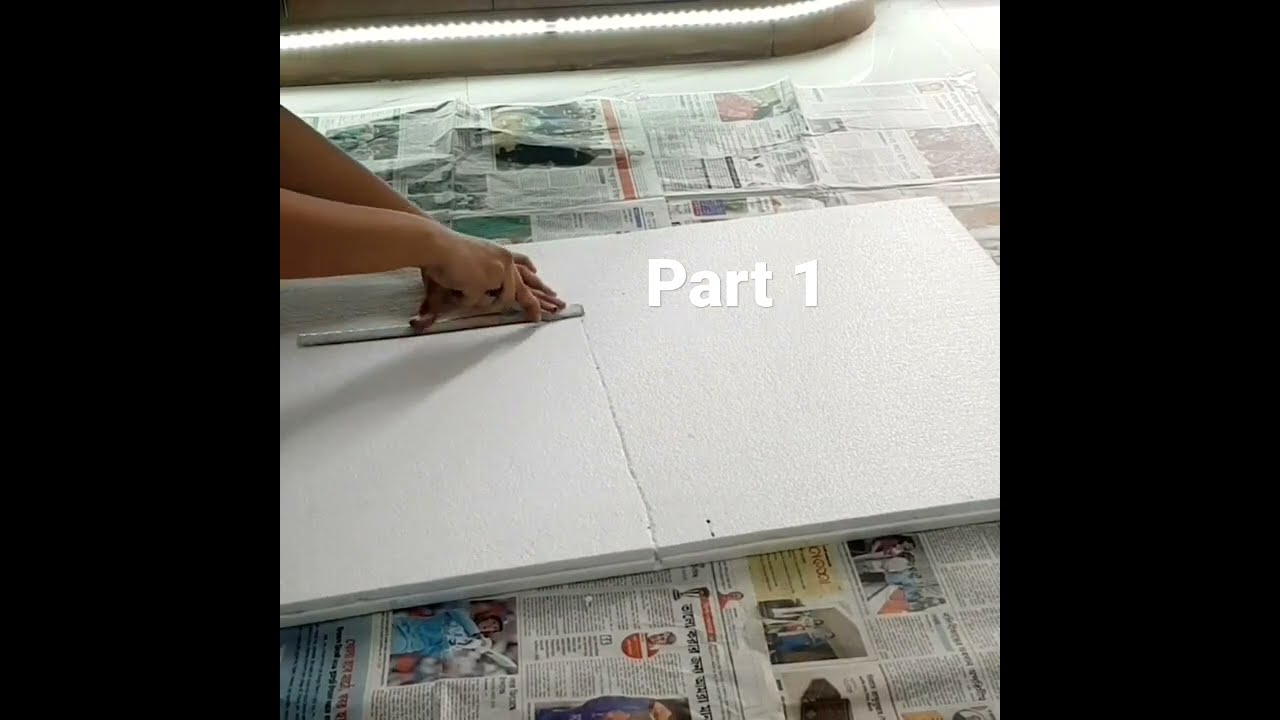The image depicts a DIY project in progress, showing a person measuring and cutting a white Styrofoam sheet using a ruler. The ruler is being pressed down by two hands: the thumb is positioned in the middle, and the other fingers are holding the top part of the ruler. The Styrofoam, approximately half an inch thick, rests on a spread of newspapers laid out neatly to manage any mess. Visible on the newspapers below the Styrofoam are various images, including sports figures playing soccer and golf. In the upper part of the frame, there appears to be a glowing item with a ring of lights, possibly corrugated aluminum, suggesting it might be another component of the project. Dominating the right side of the image is white text that reads "Part 1." The scene is well-lit with natural light, indicating it was captured during the daytime.